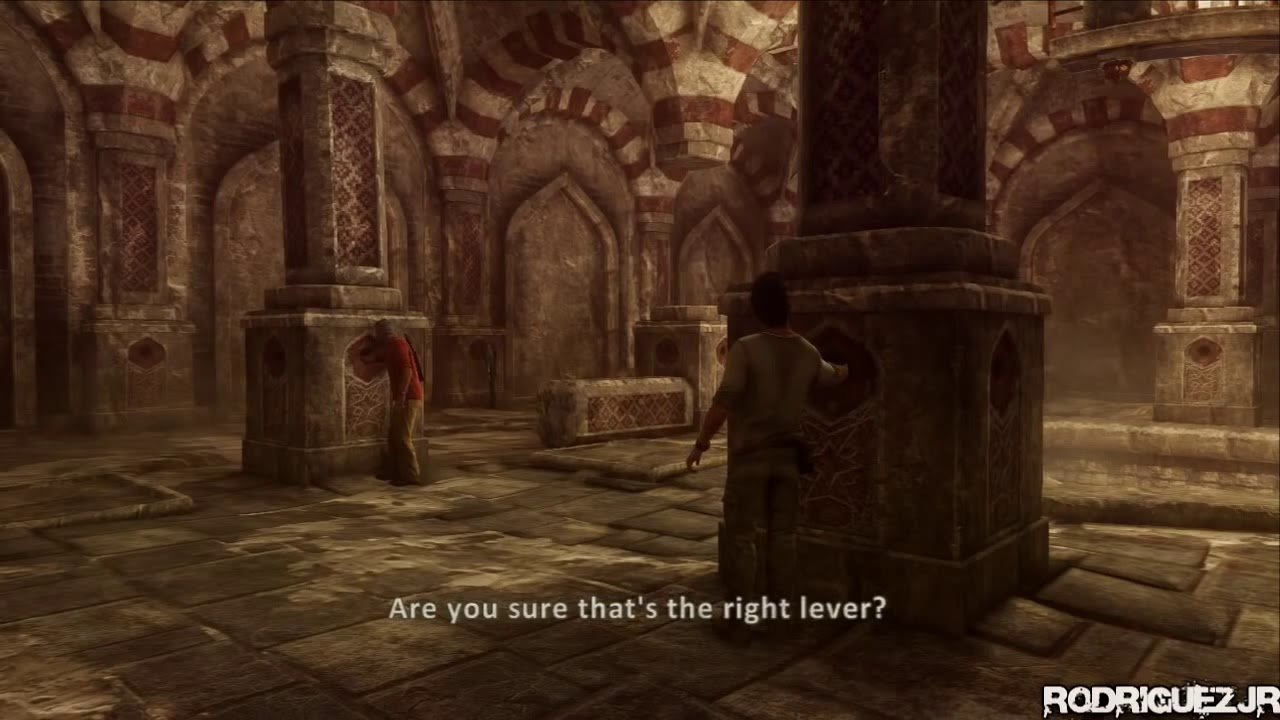This horizontal rectangular image, approximately six inches wide by four inches tall, is a detailed screenshot from the 3D video game "Rodriguez Jr.," as indicated by bold white text with black streaks in the lower right-hand corner. The scene is set within an ancient, stone-built temple, reminiscent of a Middle Eastern architectural style, characterized by sturdy stone columns, archways, and a tiled floor with large, dark brown square tiles. 

The temple's walls and entryways feature trim with alternating red and brown stripes. Central to the image are two characters. The nearest character, standing by a large stone column with his back to us, is a male wearing a brown t-shirt with visible sweat stains and brown pants. His right arm is extended to interact with a button or lever set into the column. On the left side of the scene, positioned next to another column, is an older individual with white hair, discernibly clad in a red short-sleeve shirt and khaki pants, possibly with a gun strapped to his back. This character is also focused on a similar button embedded in the column.

The setting is further enhanced by white text at the bottom of the image that reads, "Are you sure that's the right lever?" This caption adds a layer of narrative tension to the visually rich and immersive environment, suggesting the characters are in a moment of crucial decision-making within the game's plot.